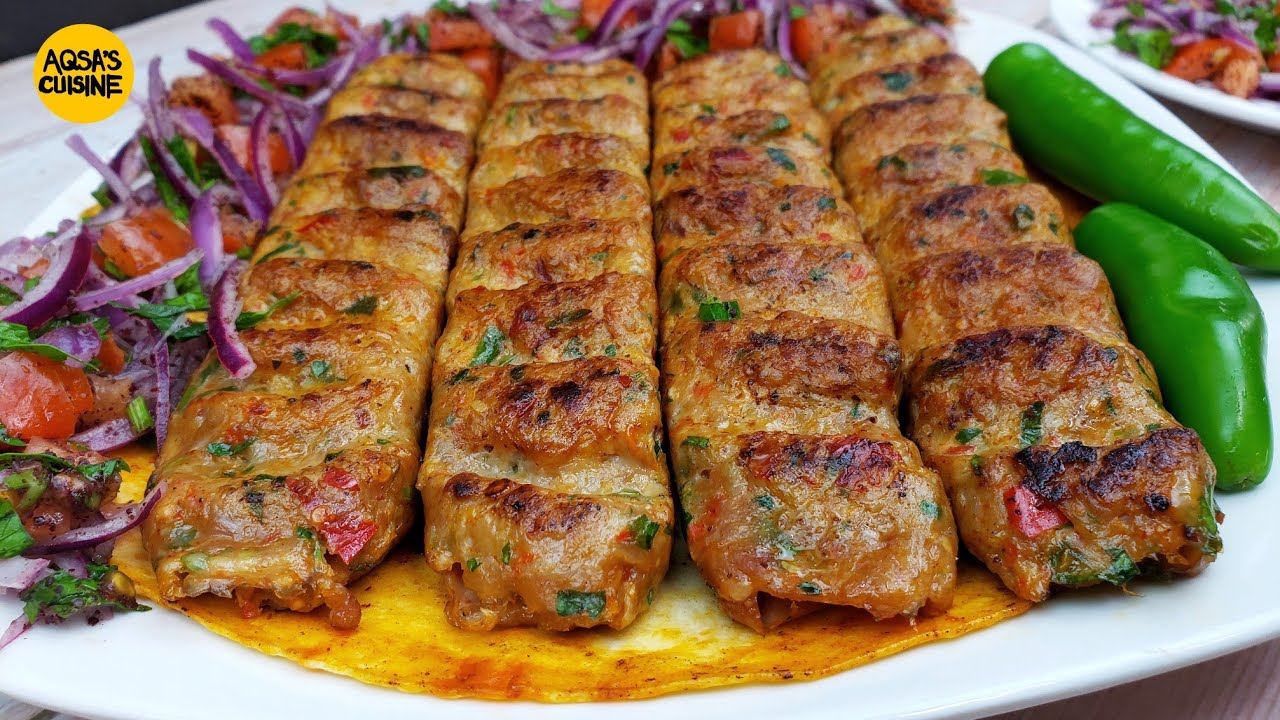This photograph features a delectable meat dish prominently displayed on a white plate, set against a brown table. At the top of the image, a gold circle with black font reads "Aqsa's Cuisine." The meat boasts a caramel-tan hue with distinctive black grill marks, suggesting it is perfectly cooked. Surrounding the meat are vibrant flakes of vegetables, including green peppers to one side and a mix of red onions and red peppers on the other. Fresh greens add a touch of color and freshness to the presentation, while an orangey juice beneath the meat hints at a tantalizing marinade or sauce. The plate's slight shadows and the gleaming surface of the green pepper reflect the high quality of the image. In the background, another plate with a similar dish is partly visible, adding a layer of depth to the composition.